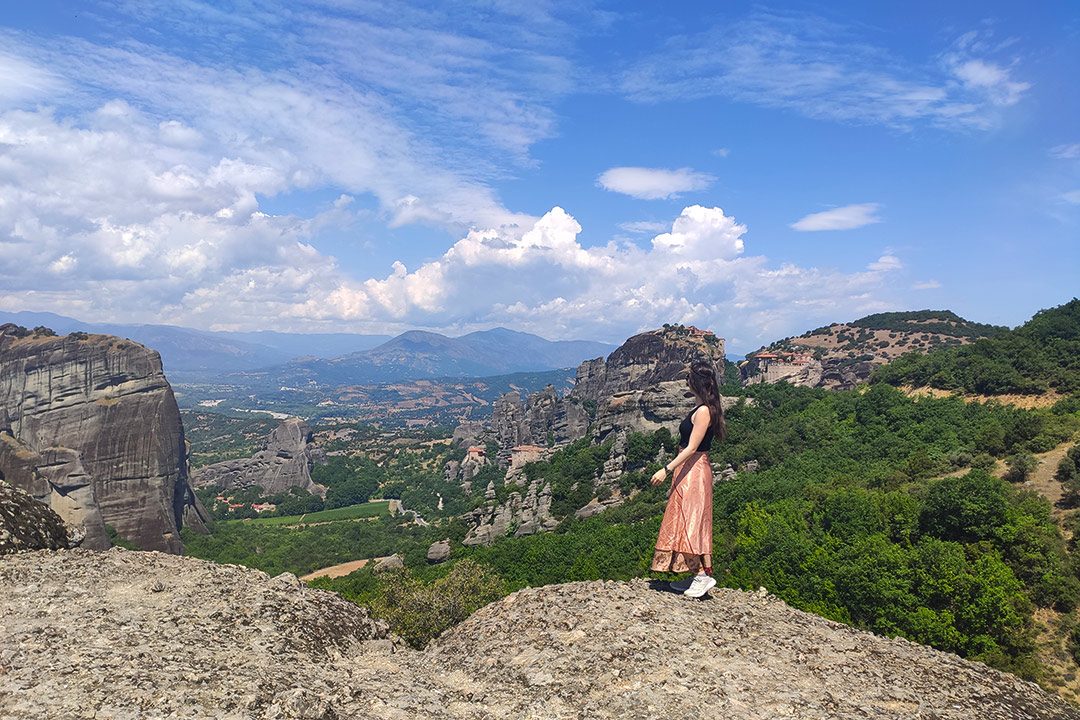In this picturesque image, a slender woman with almost waist-length wavy brown hair stands on a large rock on the side of a mountain, gazing out over an expansive landscape. She is wearing a black tank top tucked into a satiny coral pink skirt that reaches near her ankles, paired with white sneakers. An Apple Watch or similar fitness watch is visible on her wrist. The scene captures a partly cloudy day with a mix of cumulus and stratiform clouds scattered across the blue sky. The woman stands amidst lush greenery, with rocky terrain and verdant valleys spreading out below her. Far in the distance, additional mountains rise, enveloping the city nestled at the base of the hills, creating a stunning backdrop that stretches out for miles.